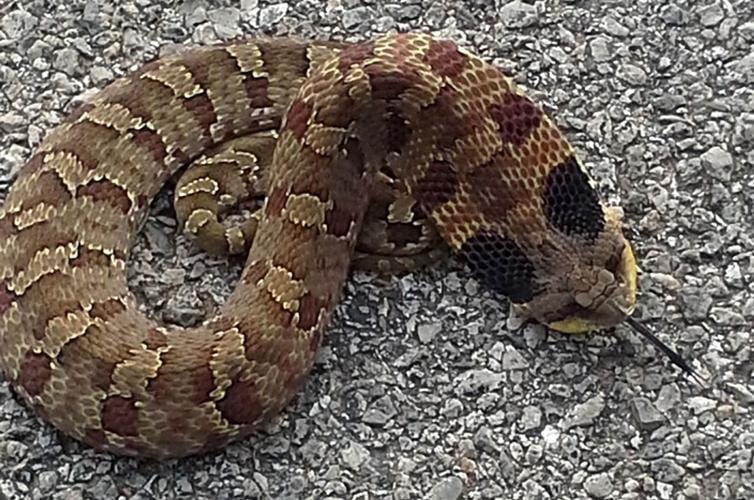The image depicts a single, multicolored snake coiled on a stone ground during the daytime. The snake's scaly body features an intricate pattern of yellow, dark red, and black stripes, reminiscent of those seen on rattlesnakes. Its head appears flattened, possibly indicating it is a member of the cobra family, capable of expanding its skin. The snake's tongue is visibly sticking out, adding to its intimidating appearance. The rocky surface beneath it consists of gray stones, and the snake is curled up tightly, obscuring where its body ends. No other elements are present in the image except for the snake and the ground.